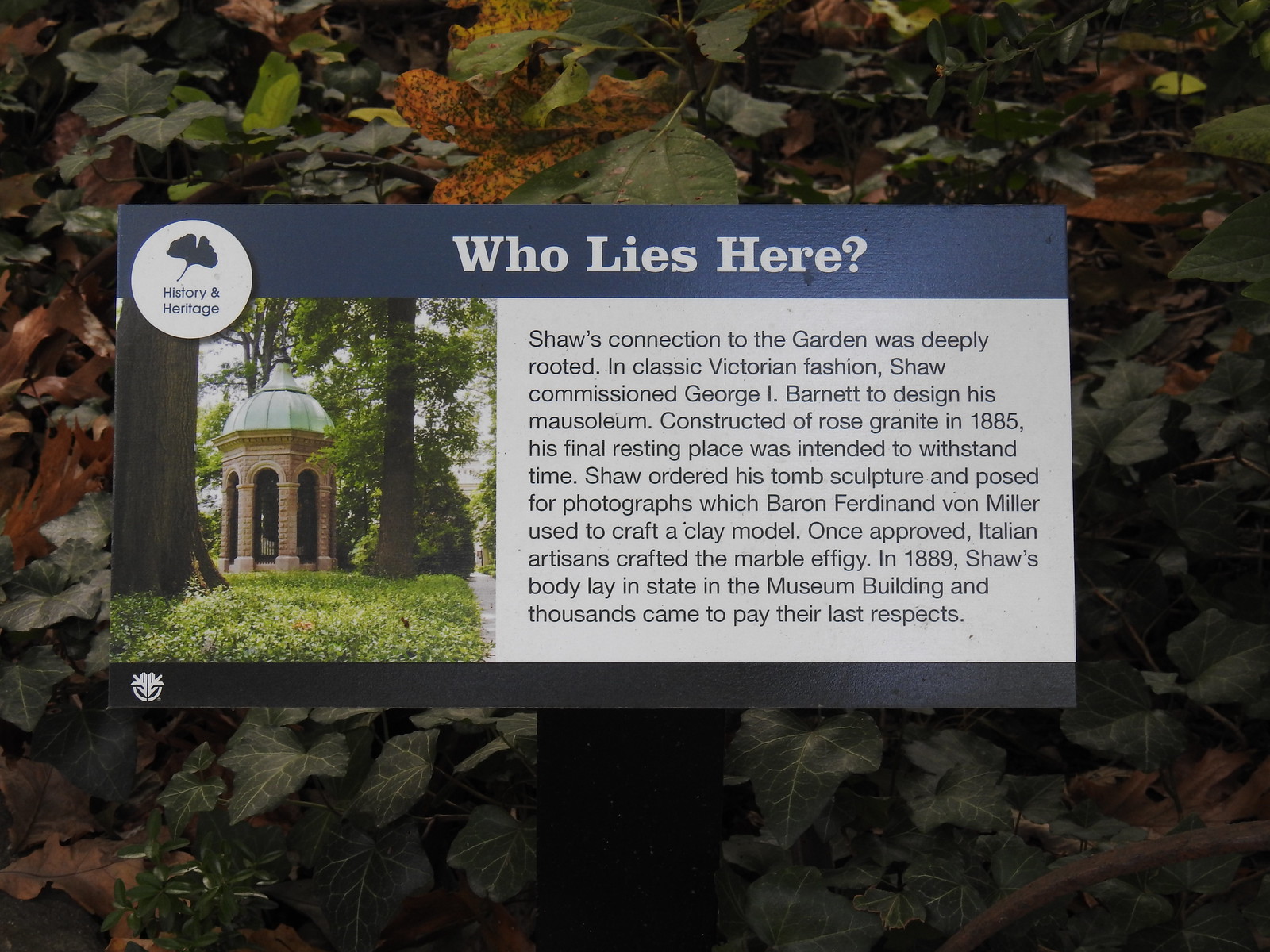The image displays a historical marker sign situated in a lush garden filled with greenery and various types of vegetation. The sign is adorned with a blue banner at the top that contains white text reading "Who lies here?" A white circle with black text proclaiming "History and Heritage" is positioned in the top left corner of the sign. 

On the left side of the sign, there is an image depicting a stone dome structure, reminiscent of a Greek temple with columns, nestled in a forest pathway. The central portion of the sign features detailed text explaining the significance of Shaw's connection to the garden. The text mentions that in the classic Victorian style, Shaw commissioned George I. Barnett to design his mausoleum, which was constructed out of rose granite in 1885. The mausoleum was meant to endure through time.

The narrative goes on to describe that Shaw himself organized the tomb sculpture and posed for photographs, which Baron Ferdinand von Miller used to craft a clay model. Once approved, Italian artisans sculpted the final Marble Effigy. In 1889, Shaw's body was laid in state in the museum building, where thousands of people came to pay their last respects.

The sign is mounted on a black stand with a black banner below it, and the ground around it is covered with various shades of green and brown leaves, adding to the historical and natural ambiance of the garden setting.